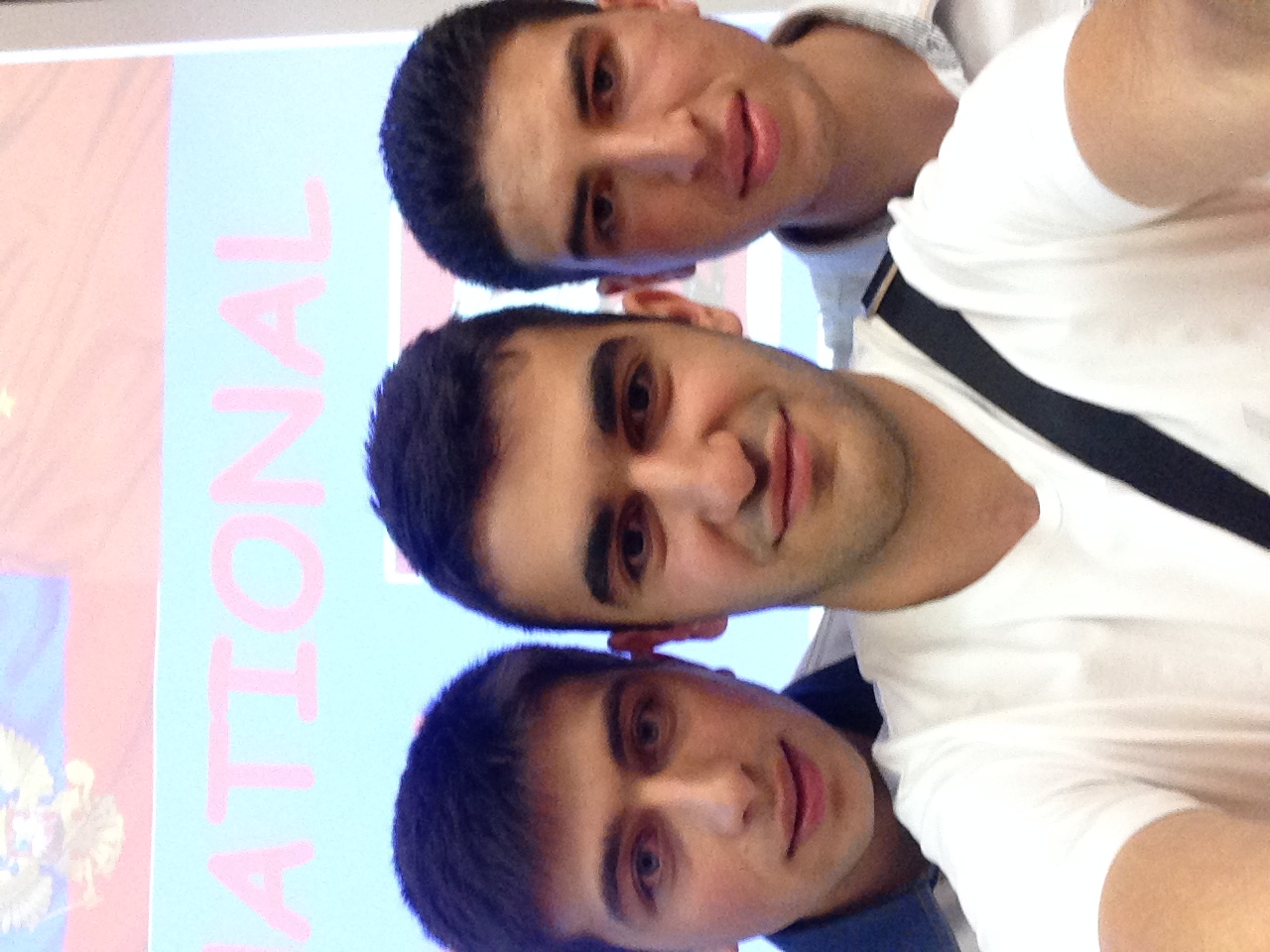The photo features three young men, likely in their early 20s and of Indian descent, standing close together with the man in the middle holding the camera for a selfie. Each has very dark, short black hair, bushy eyebrows, dark eyes, large noses, and thick lips, making them strikingly handsome. The man in the center, in the forefront, is easily the most visible, sporting a white v-neck t-shirt and a black shoulder bag strap. He has a half-smile and looks straight at the camera. To his right, you can just glimpse the face of another young man, identifiable by his short black hair and the blue collar of his shirt. On his left, another young man, also with short black hair, is partially visible from the neck up, wearing a light-colored shirt and also looking forward. Behind them is a banner with a pink top and the word “International” in pink letters on a green background, hinting at a student exchange program. The banner is partially obscured by their heads and extends out of the frame at the top.